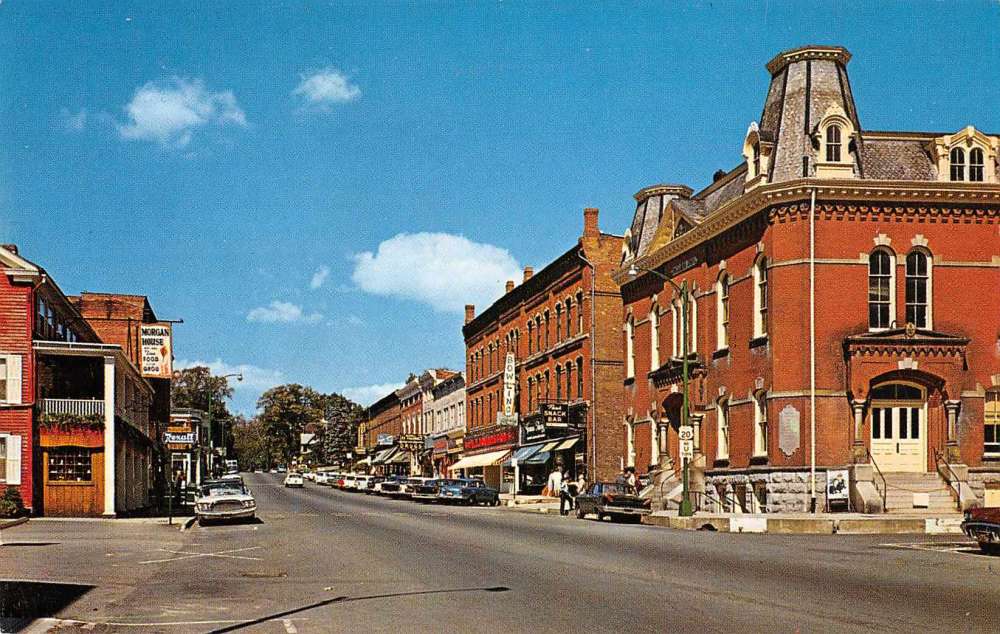The photo captures a picturesque intersection in what appears to be the business district of a small American town from the 1950s or early 1960s. The scene is set under a partly cloudy sky with blue and white tones. The main street, lined with two and three-story brick buildings, includes storefronts and possibly a courthouse or government building on the right side. A sign for "Morgan House" is visible on one of the buildings, while another features a bowling alley and bar. A white car is seen traveling down the road, opposite to several parked vehicles, including a distinctive red or brown car from the 1950s with two headlights on each side. The street has visible white markings and crosswalks, with a prominent highway sign indicating U.S. Route 20 and a "No U-turn" directive. Pedestrians are scattered along the sidewalks, with colors from their clothing adding splashes of blue, white, brown, orange, red, and black. The street extends towards a tree-lined horizon, slightly curving over the crest of a hill, giving the town a quaint and nostalgic charm.